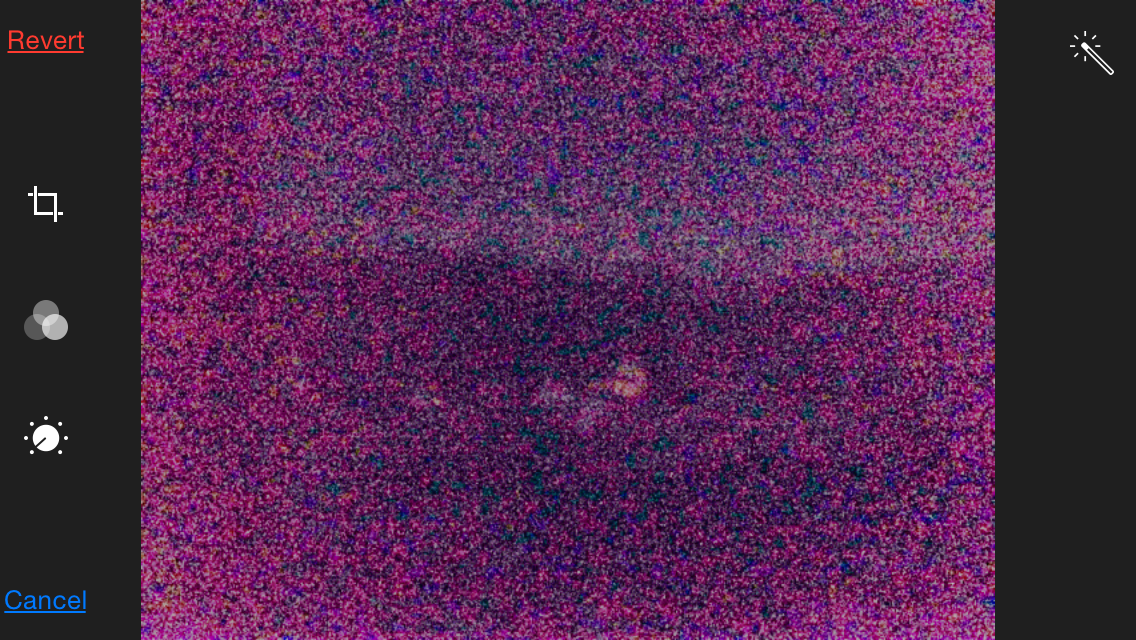In this pixelated image, the horizon is adorned with an array of lighting sources that create a mystical ambiance. The sky transitions through a palette of purples, light browns, oranges, and hints of red, creating a mesmerizing blend of hues. The pixelation enhances this ethereal mosaic, adding a unique texture to the visual experience. 

The left-hand side of the image is dominated by various image editing icons. At the top, a red "revert" button is prominently displayed, followed by a cropping symbol. Below these, three overlapping circles likely represent contrast or hue adjustments. Additional symbols, including one that is unfamiliar, diversify the options further. Towards the bottom left, a blue, underlined text labeled "Cancellum" is visible.

In the upper right corner, an icon resembling a wand with ticks near its end adds a touch of whimsy to the editing panel. Flanking the image are black columns, and the background remains steadfastly black, framing the image and editing tools in a stark contrast that accentuates the vibrant colors of the horizon. The composition invites viewers to both appreciate the image and imagine the possibilities of its transformation through editing.